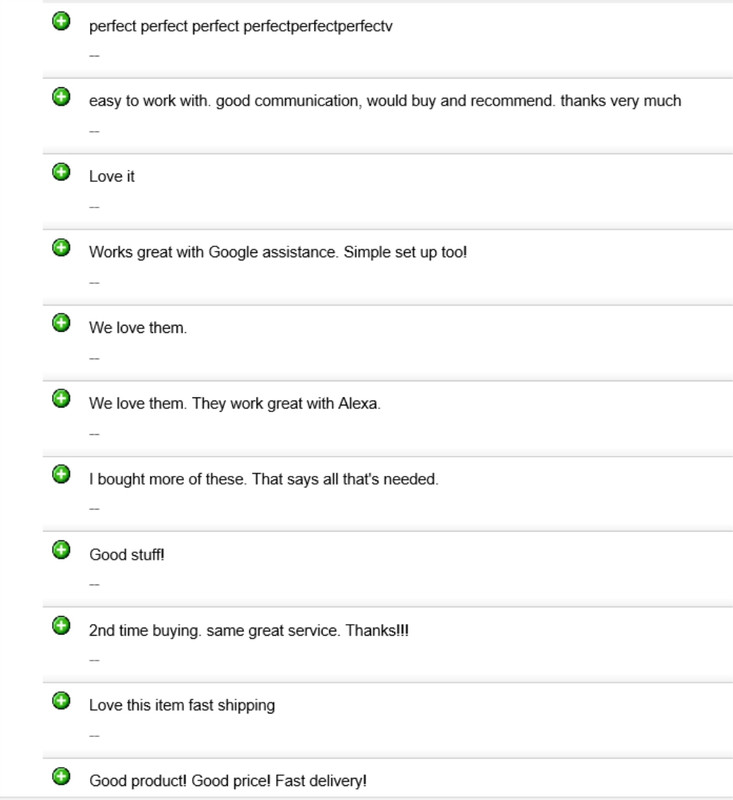This screenshot showcases a list of product reviews, presented in a clean, minimalistic format. The page features a white background with black text and is divided by thin gray lines, giving it an organized, tabular appearance. On the left side of each review entry, small green circles with white plus symbols inside them are displayed. All reviews listed are positive, with recurring phrases such as "perfect," "easy to work with," and "good communication." Other notable comments include compliments like "would buy and recommend," "works great with Google Assistant," "simple to set up," and "great service." Reviews also mention fast shipping, good product quality, and reasonable prices. Despite the simplicity of the reviews and absence of detailed user information or specific product identity, the overall sentiment is distinctly positive. The page layout and color scheme are straightforward, focusing solely on the content of the reviews.